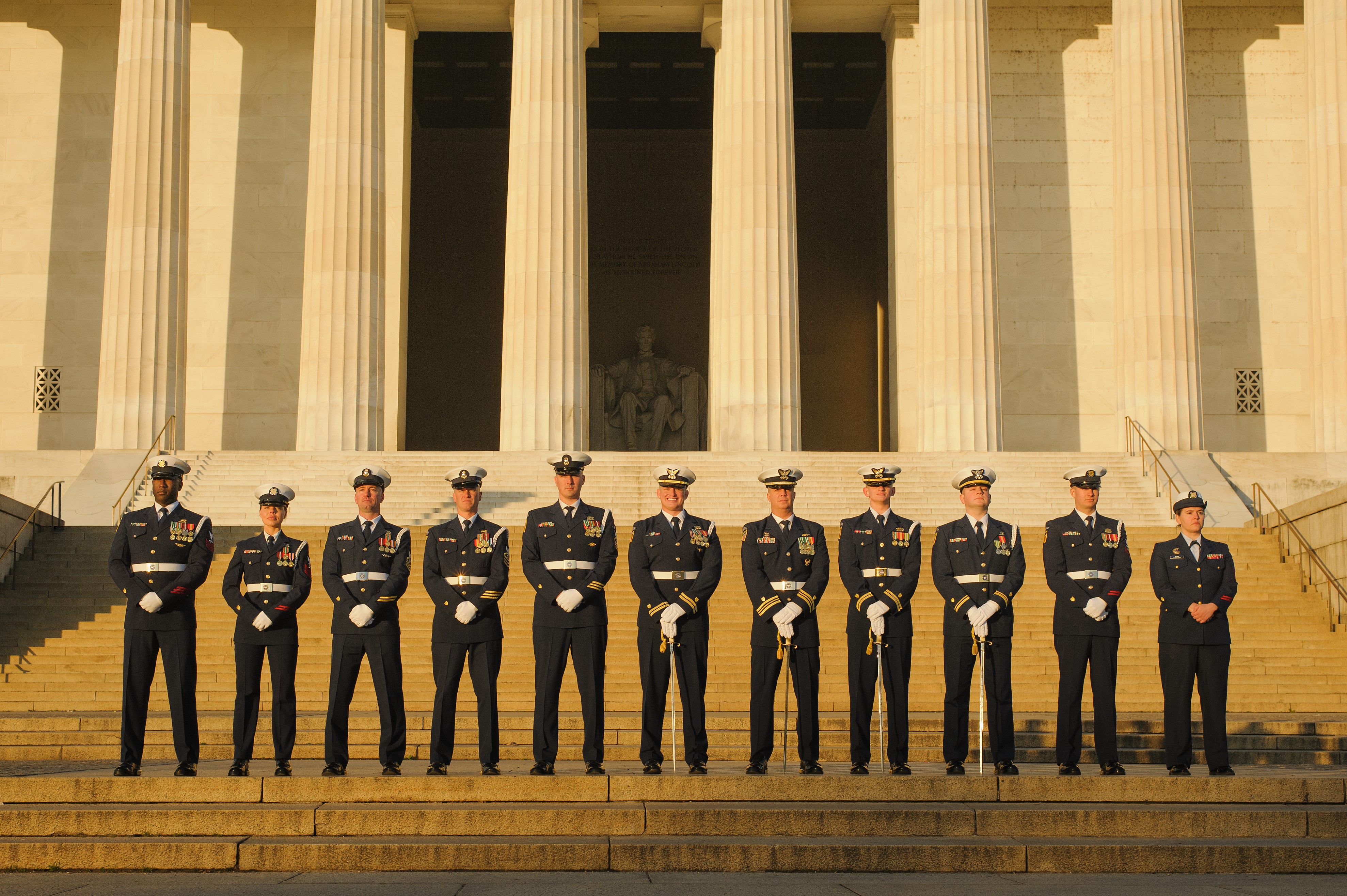This photograph captures 11 service members standing side-by-side in uniform on the steps of a large white building with prominent columns, which appear to be marble-like. Behind them in a recessed area is a sculpture of Abraham Lincoln, partially shrouded in darkness. The service members, a mixture of men and women, are dressed in very dark blue uniforms with white belts and gloves, except for the last person on the right who is not wearing gloves. They all wear white caps with blue bills, and their cuffs feature gold embroidery along with various patches on the left sides of their uniforms. About four of them hold long, thin foil swords pointing straight up from the ground to their hands. Some members are smiling while others maintain a serious expression, and the sunlight gives the steps a golden hue.